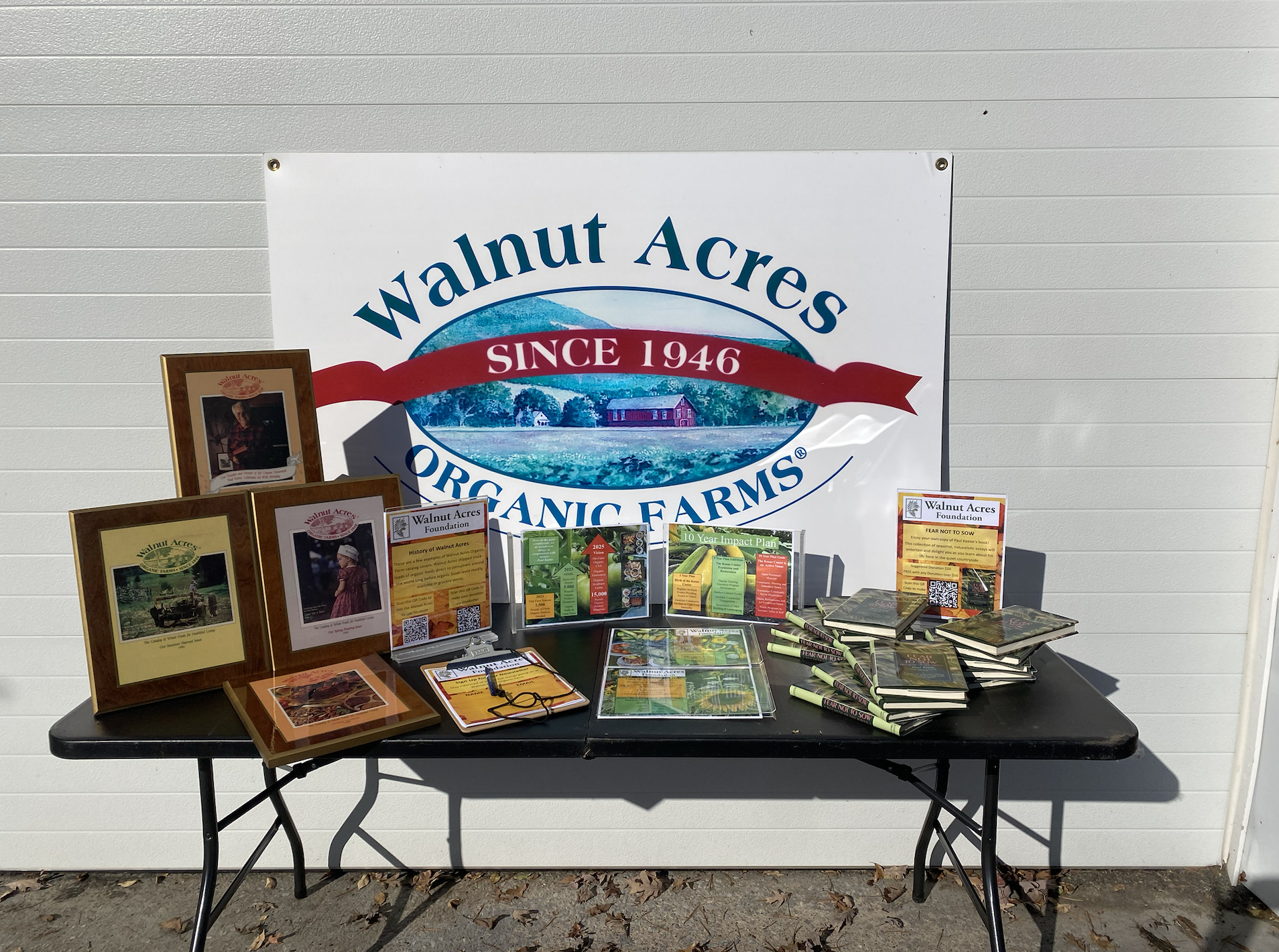The image features an outdoor display set against a wide, white-paneled door, likely a garage or storage door. A prominent white sign is pinned to the wall, announcing "Walnut Acres Organic Farms" in blue font, with a red banner reading "Since 1946," accompanied by an illustration of a red farmhouse with a slanted gray roof among trees. Below the sign is a black wooden-style fold-out table, approximately six to eight feet long, typically used for events or conferences. The table is neatly arranged with various promotional and informational items. On the right side, there are scattered books, while the center holds cards with information, possibly a sign-in sheet on a clipboard. To the left, there are photographs in wooden frames. Additionally, two stand-up signs read "Walnut Acres Foundation," with text too small to make out. The setup appears designed to showcase the history and mission of Walnut Acres, likely for an event or public presentation.